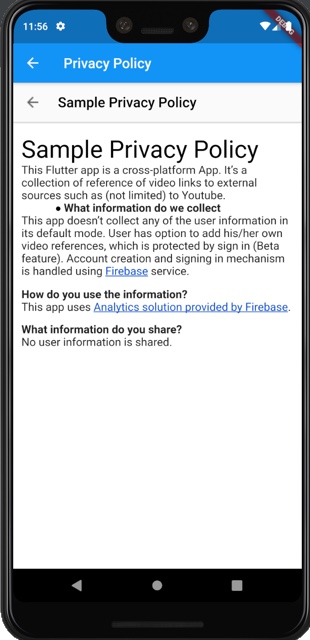A detailed descriptive caption for the provided image content could be:

"A screenshot of a website's privacy policy displayed on a smartphone. The screen is oriented in portrait mode, showing a timestamp of 11:56 at the top left and a nearly full battery indicator at the top right. Adjacent to the battery icon, a red 'debug' label is diagonally overlayed. The top of the screen features a blue banner with the text 'Privacy Policy' in white. Directly below, a gray banner reads 'Sample Privacy Policy.' The main body begins with the bold heading 'Sample Privacy Policy,' followed by a paragraph in smaller text. The text mentions that the app in question is the 'Flutter app,' a cross-platform application that provides a collection of reference video links to external sources, including but not limited to YouTube. It further states that the app does not collect any user information in its default mode."